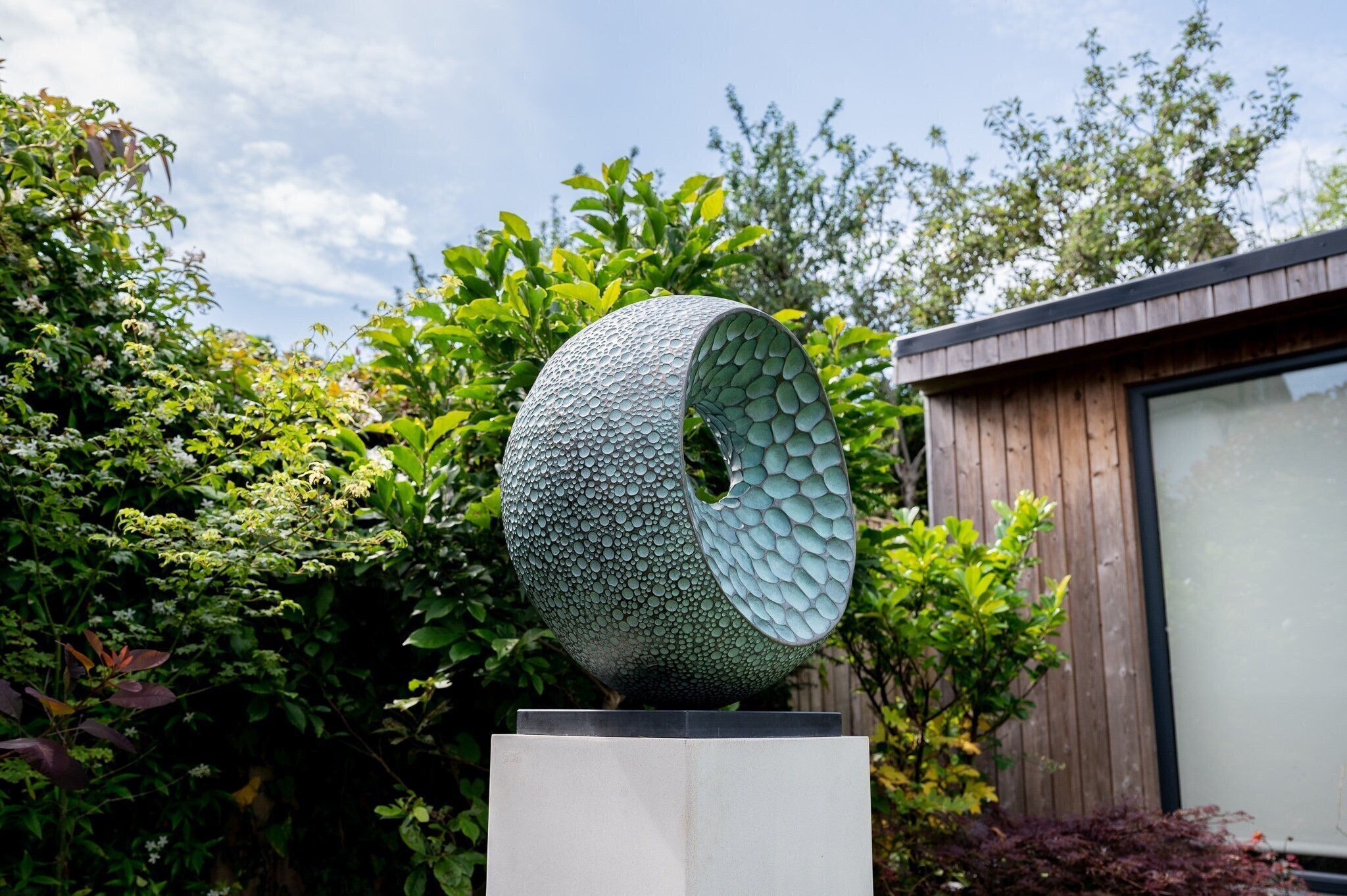The photograph captures a striking outdoor scene featuring a sculpture prominently placed in the center. The sculpture, a thick circular ring with a textured, pockmarked surface, stands about two to three feet high and wide, with a circular hole at its center. The sculpture has a light green-turquoise hue, reminiscent of oxidized metal. It is mounted on a square, concrete pedestal designed with a recessed black square display, elevating the artwork about three to four feet above the ground.

The background reveals a lush garden setting, with green bushes and some dark red foliage. To the right of the image, there is a house with a wooden exterior and a large, reflective window that catches the surrounding greenery. The scene is bathed in natural light from a blue sky dotted with a few puffy white clouds, capturing the essence of a pleasant day.